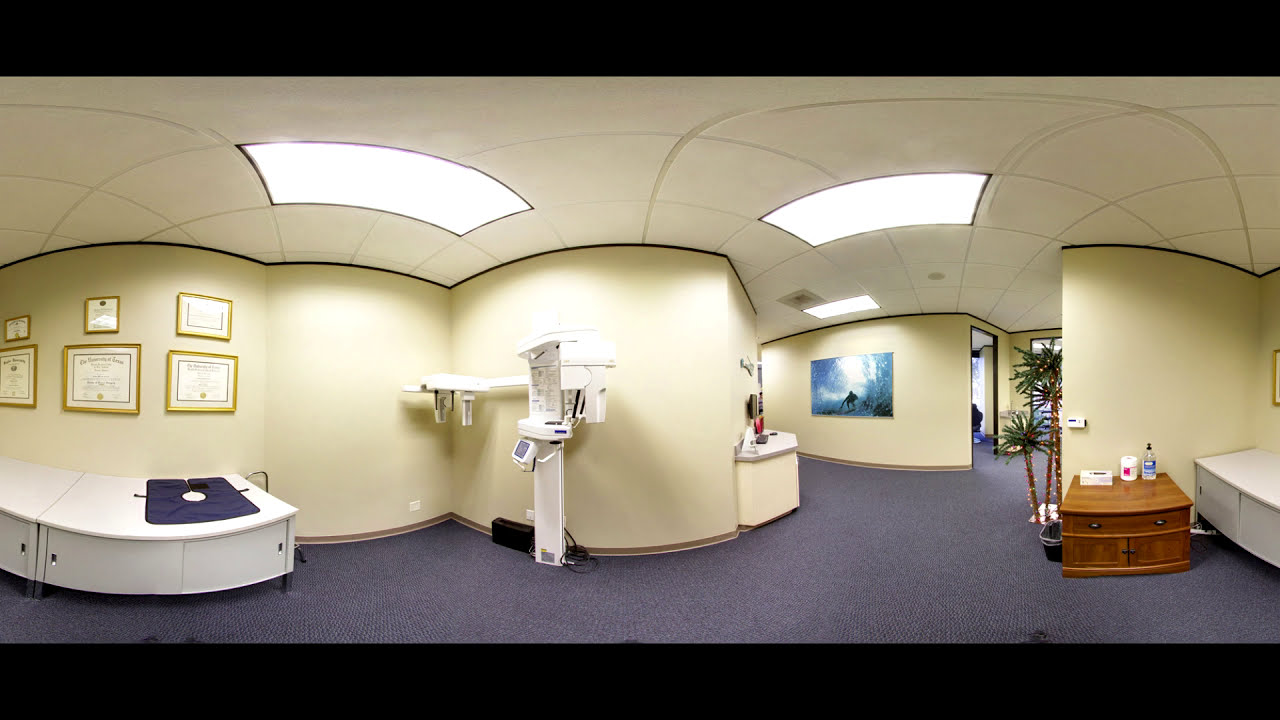This image captures a doctor's office setting, viewed from a fisheye lens perspective which distorts the edges, giving the room a stretched and wavy appearance. Dominating the center of the room is a high-tech piece of medical equipment, possibly a scanner. Surrounding it are various furnishings and tools, including short cabinets on the left and a dresser-like storage area on the right. The area to the right also holds what seems to be hand lotion and a decorative palm plant. 

The walls are adorned with professional credentials and artwork, contributing to the scholarly and aesthetic appeal of the space. The office ceiling features distinctive, warped tiles, while the floor is covered with a dark gray carpet that extends throughout the room. The setting is accentuated by excellent lighting, likely from overhead lights visible in the image. 

The front desk is situated towards the top right corner, balancing the well-organized layout of the room. The color palette is varied, including shades of black, purple, white, brown, red, blue, green, and yellow. There is no visible text in the image, and the room is devoid of people, emphasizing a tranquil and professional medical environment.